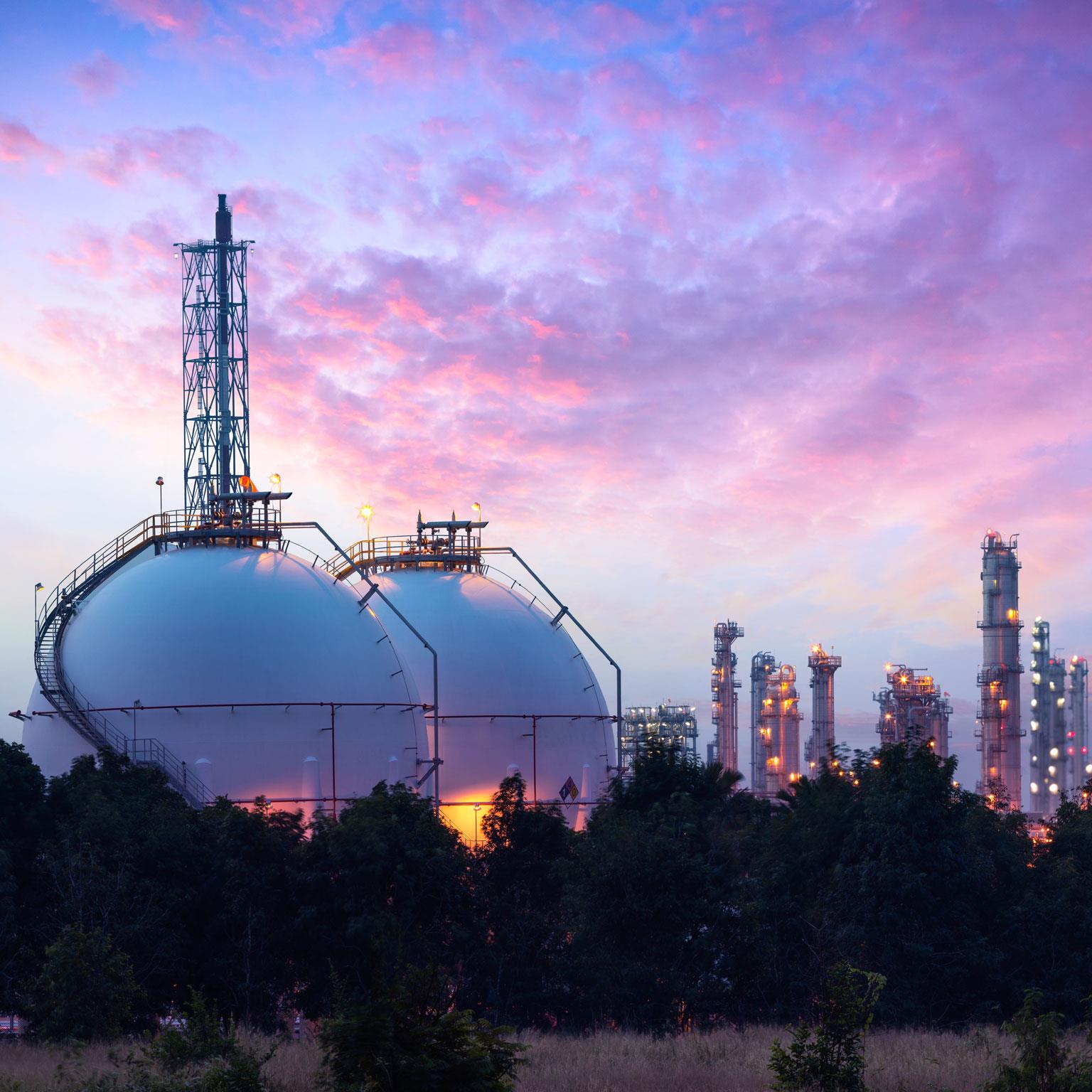This is a highly detailed, square-shaped photograph of an industrial facility, captured during twilight hours, either at dawn or dusk. The sky exhibits a beautiful gradient of blue, red, purple, and pink hues, adorned with scattered clouds, suggesting the sun is either rising or setting. In the foreground, brown grass and green shrubs, approximately 10 feet tall, frame the image. The centerpiece on the left side consists of two enormous, white, spherical storage tanks, each around 50 feet tall, encased in intricate scaffolding, piping, and metal supports. A stairway winds up to the top of these globes, possibly storing chemicals or gases. Towards the right side of the frame, several metal towers, including about nine lit towers extending up to 100 feet tall, are visible, equipped with lights, ladders, and additional industrial fittings. The overall scene, while illuminated by the picturesque colors of the sky, clearly depicts an industrial facility, likely an oil refinery or similar plant, set against the serene backdrop of a striking twilight.